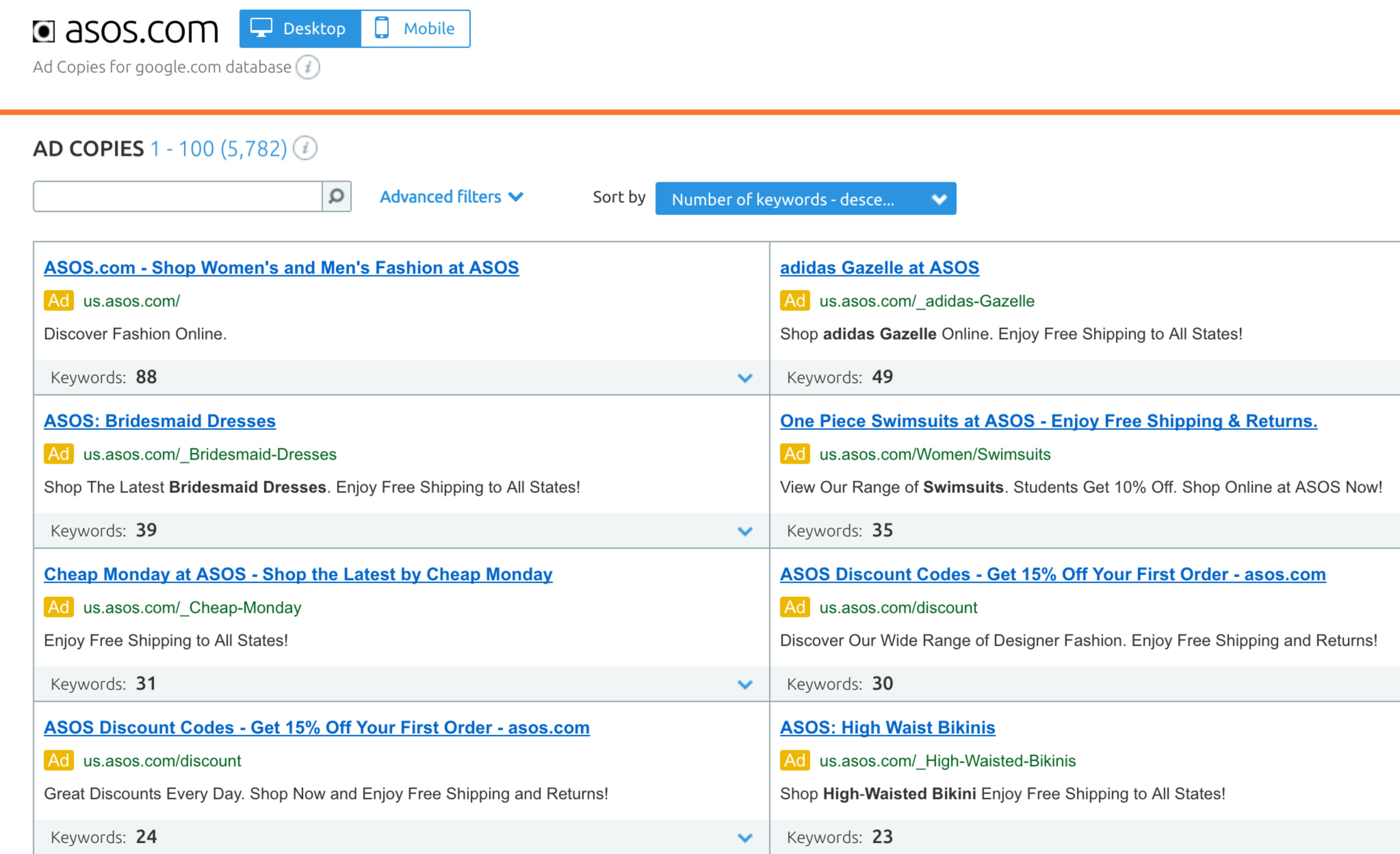This image appears to be a screenshot from the ASOS advertising interface within the Google Ads platform. The interface offers the option to switch between desktop and mobile ad views. 

On the page, there's a prominent toggle switch allowing users to select between desktop and mobile views. The desktop option is highlighted in blue with white font, while the mobile option is in white with blue font. The toggle switch is designed as a long rectangle divided in the middle, featuring icons of a desktop monitor on the left and a cell phone on the right.

Above the toggle switch, there's an orange line accompanying the text "Add Copies: 1-100 (5,782)", indicating the total number of ad copies available. Adjacent to this text, there is an 'eye' icon within a gray circle that likely serves as a visual representation of visibility or preview functionality.

Below this section, there's a search bar characterized by its white color, gray outline, and a gray magnifying glass icon. Next to the search bar is an "Advanced Filters" option with a downward menu symbol, indicating expandable filter options. Following this, there is a text for "Sort by number of keywords - decrease," accompanied by a dropdown menu.

On the left side of the interface, there's a list of ad copies. The first ad copy is for asos.com, with the text: "Shop women's and men's fashion at ASOS. Discover fashions." This ad uses 88 keywords. The second ad copy in the list is for "asos bridesmaid dresses," featuring the text: "Shop the latest bridesmaid dresses, enjoy free shipping in all states," and utilizes 39 keywords.